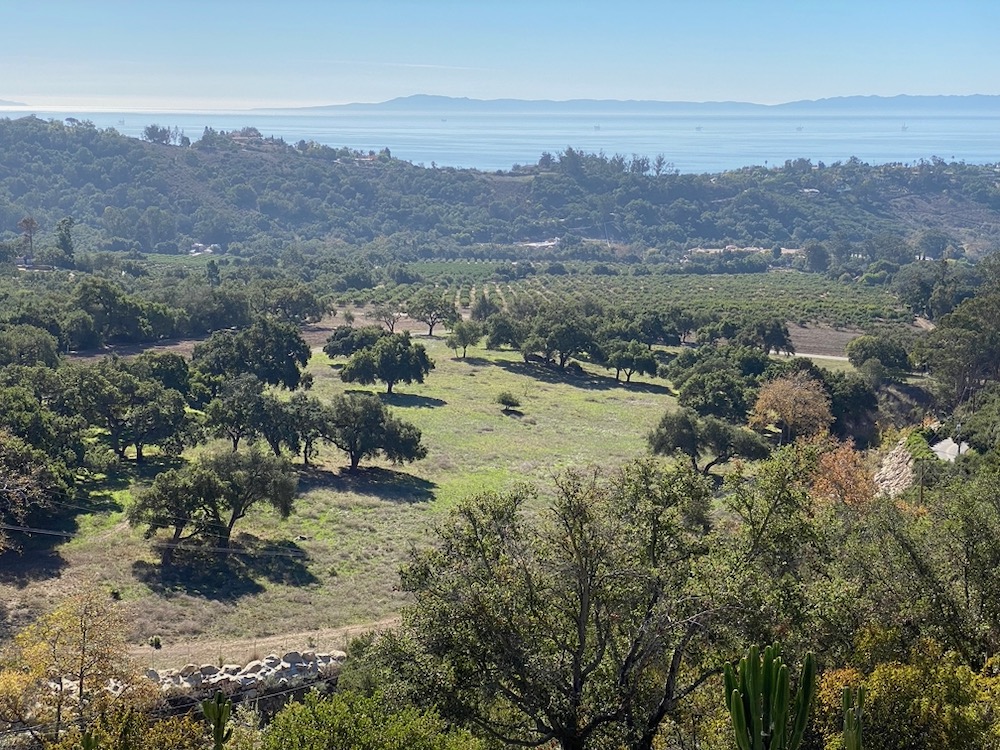This wide-angle photograph captures a stunning daytime landscape featuring a serene harmony of hills, valleys, and an ocean in the far distance. The light blue sky, which almost mirrors the hue of the ocean, stretches across the background. A silhouette of dark brown mountain ranges sits just below the sky, with a glimpse of blue water peeking through. Forward from the mountains, the hills are densely covered in dark green trees and shrubbery. 

In the foreground, the vibrant, open valley displays a mix of dark and light green grasses interspersed with tan patches. To the right, a small orchard with neatly ordered rows of green trees stands out against the backdrop. A winding one-lane dirt road lined with rocks wraps around the grassy expanse, leading the eye through the composition. In the bottom right corner, a cluster of trees, some with dead leaves, and a cactus add to the textural variety of the scene. The Sun is high above, casting clear shades beneath the various trees and bushes scattered throughout the area. Some bushes in the foreground exhibit hues of yellow and brown, providing a rich color diversity to the landscape.